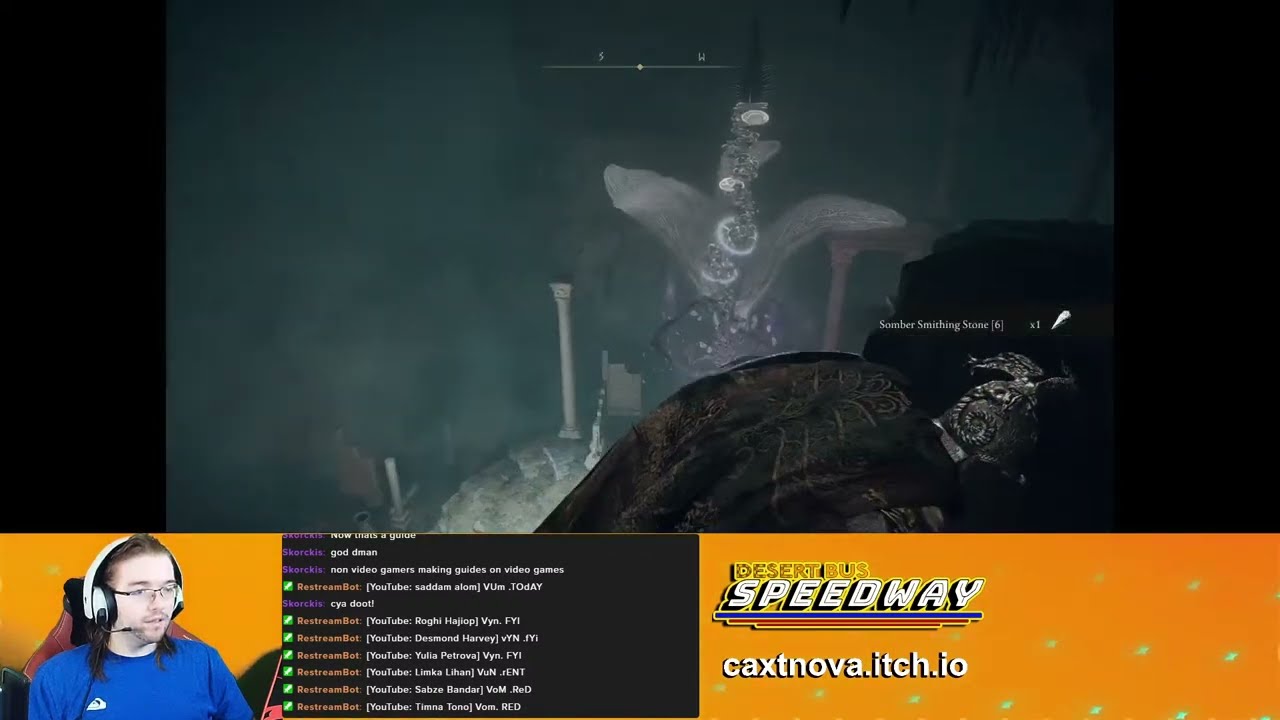In this image, a white male streamer with long brown hair, wearing glasses, and dressed in a blue Quicksilver shirt sits in front of an orange background, broadcasting a video game. He’s seated in a white gaming racing chair, and wears a white headset with a microphone positioned near his mouth. The main part of the image shows gameplay from "Elden Ring," featuring underwater scenes, pillars, and mountains, along with a character wearing a green cape adorned with gold designs. On the bottom left of the screen, the streamer’s facecam is visible. To the right of this, the Twitch chat window displays usernames in purple and white text. An orange section on the lower right features the "Desert Bus Speedway" logo in white and orange, with a blue and red border beneath it, and the text "CAXTNOVA.itch.io" below white stars on an orange background. Black bars frame the main broadcast image on either side.